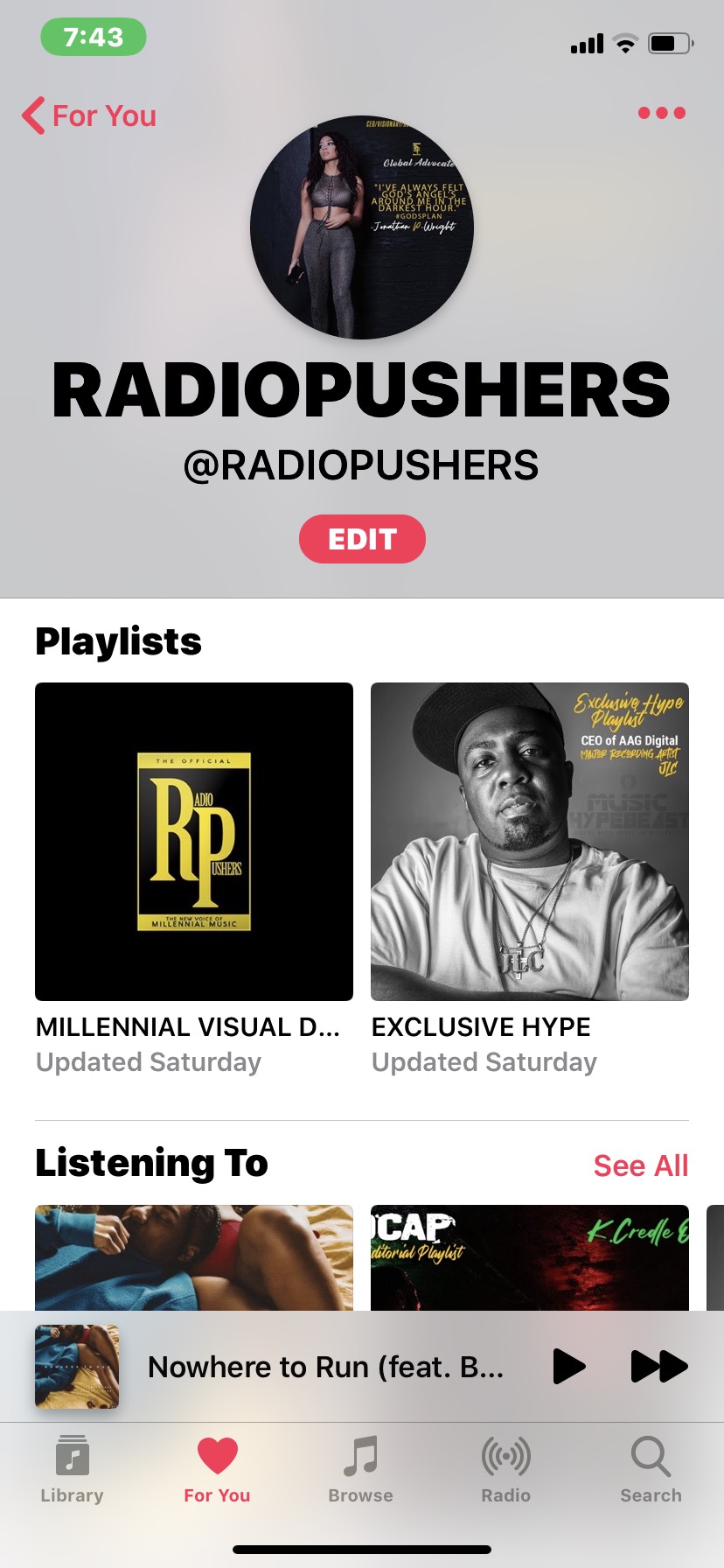The screenshot, captured from a cell phone, displays the device's status bar at the top. It is 7:43 AM or PM, the mobile signal shows two out of three bars, the Wi-Fi connection is at two out of three bars, and the battery is at 50%. Below the status bar is a gray square. In the top left corner of this gray square, there is a red "4U" icon with an arrow pointing left. On the top right of the gray square are three red dots. 

In the center of the gray square is a circular image displaying an album cover. The cover features a woman wearing jeans, standing against a black wall. Below this image, "Radio Pushers at Radio Pushers" is written in bold black font. Underneath this text, there is a green button with the word "Edit" in white font. 

Following the gray square, the background of the page turns white. At the top of this section, "Playlists" is written in black font. Below "Playlists" are two squares side by side. The left square is black with a yellow square inside it carrying the letters "RP." This square is labeled "Millennial Visual D, updated Saturday." The square on the right is gray and features an image of a man of African descent wearing a black baseball cap and a white t-shirt.